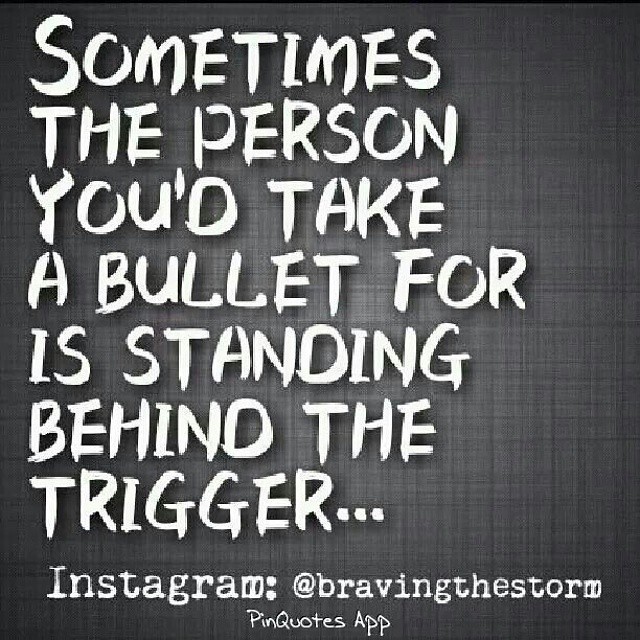The image appears to be a poster-like Instagram or Pinterest post featuring a thought-provoking quote. The background is a dark charcoal gray, resembling fabric, with a subtle checked pattern and a gradient lighting effect that radiates from the center, making it slightly brighter in the middle and darker at the edges. Across the center of the image in large, all-caps white font with a paintbrush brushstroke style, the quote reads: "Sometimes the person you'd take a bullet for is standing behind the trigger..." Below this quote, the text cites the handle "@braving the storm" on Instagram, followed by the source, "pin quotes app." The overall aesthetic is dark and moody, with the white, slightly frazzled lettering providing a stark contrast against the somber background.